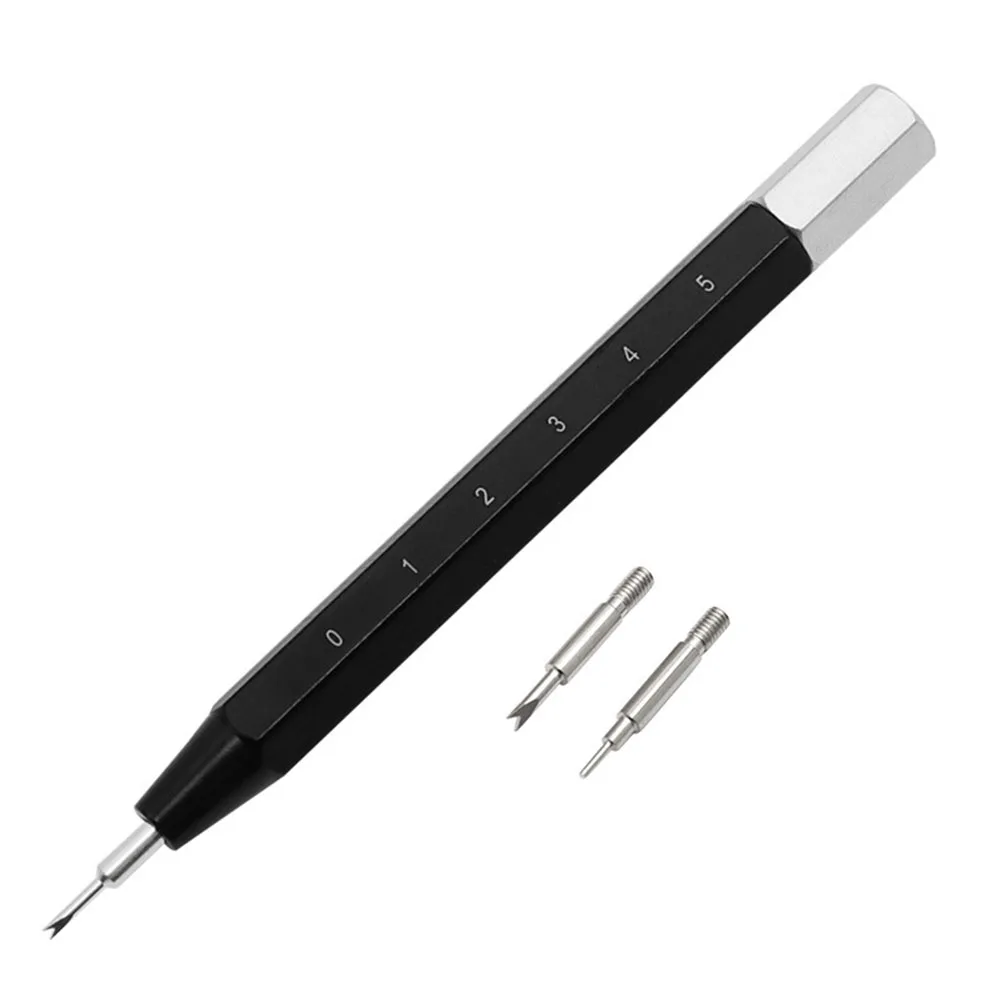The image showcases a detailed, sleek instrument resembling a pencil but primarily black with metallic silver accents. The upper end features a silver, metal-like segment similar to where an eraser would be on a pencil. The body, which is black, has numbers 0 through 5 evenly spaced, likely about half an inch apart if this were actual size. The pointed lower end of the instrument is equipped with a two-pronged, forked attachment that resembles a snake's tongue, also metallic silver. To the right of the main instrument, there are two additional replaceable heads—one shaped similarly with a forked design and another resembling the tip of a mechanical pencil, both made entirely of silver metal, potentially stainless steel. This setup suggests the instrument is a versatile tool with interchangeable heads, suitable as a mechanical or precision device. This image possibly serves an advertising purpose, highlighting the tool's multifunctional design.